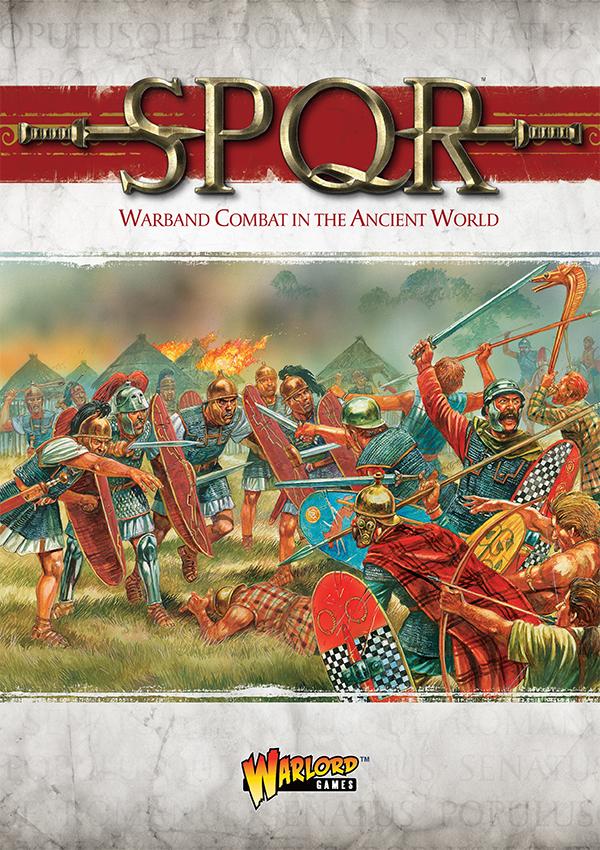The image portrays the front cover of a book or game set against a dirty white, grayish background adorned with faint, indistinguishable letters. At the top, a prominent red banner features the tarnished gold letters "S-P-Q-R," flanked by swords piercing through the 'S' and 'R'. Below, text in red reads, "Warband Combat in the Ancient World." The central illustration depicts a chaotic battle scene with Viking or Roman warriors clad in skirts and capes, wielding red shields, swords, and bows and arrows. The warriors, some wearing gold helmets with red plumes, are engaged in fierce combat on a grassy field, while the background reveals mountains and flaming structures. At the bottom, "Warlord Games" is written in orange letters.